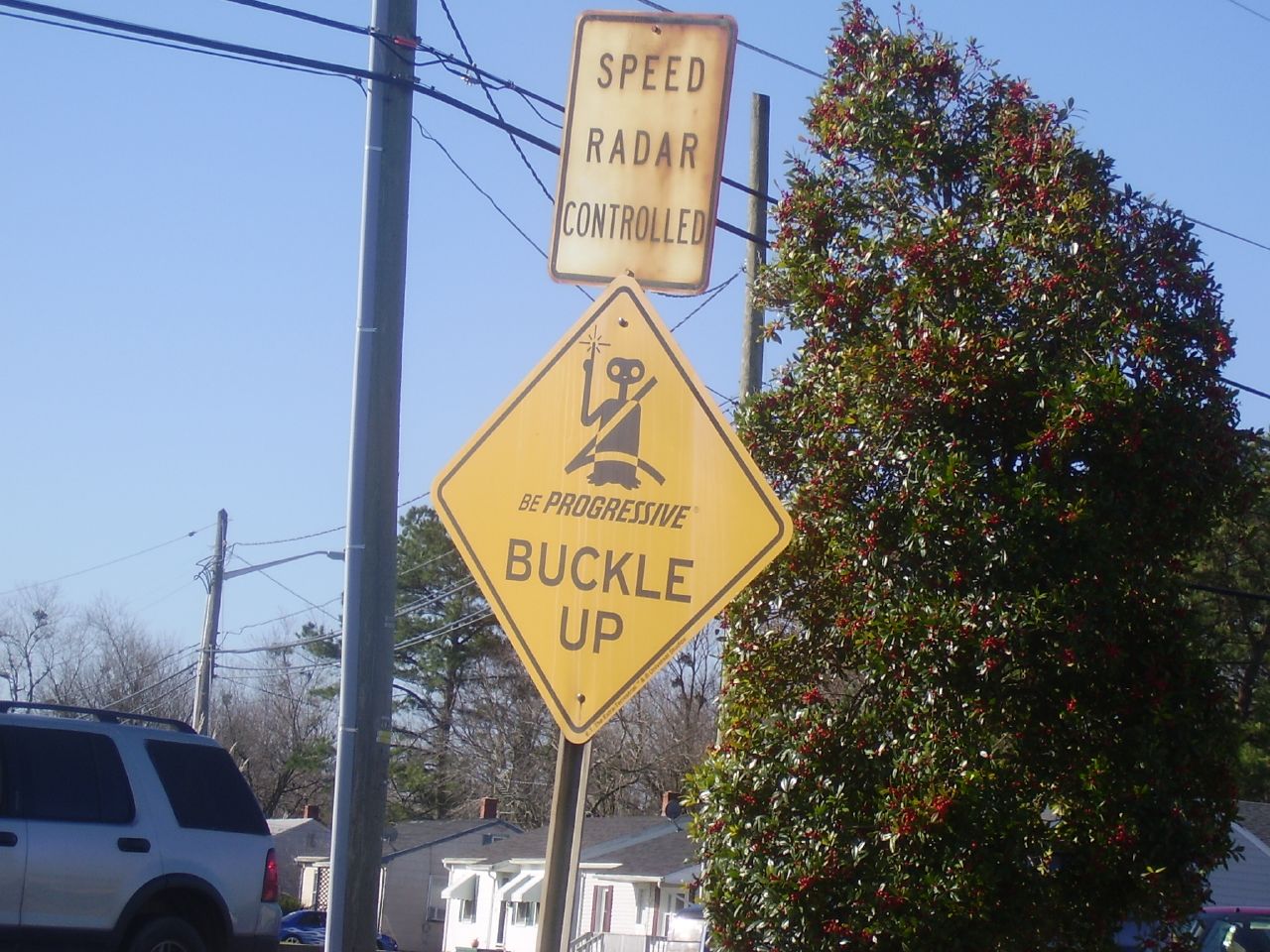In the outdoor color photograph, a tree with predominantly green leaves and some red flowers stands prominently on the right side, suggesting early autumn. Directly in the center is a gray pole featuring two road signs: the top rectangular sign reads "Speed Radar Controlled" with a rusted edge, and the yellow diamond-shaped sign below it shows an icon of a person wearing a seat belt, accompanied by the words "Be Progressive, Buckle Up." Power lines extend from a pole on the left side across the top of the image. On the bottom left, a silver car with black windows and wheels is parked, and another blue car faces a row of one-story white houses with gray roofs in the background. The scene is bathed in the clarity of a blue sky, capturing a typical suburban setting.